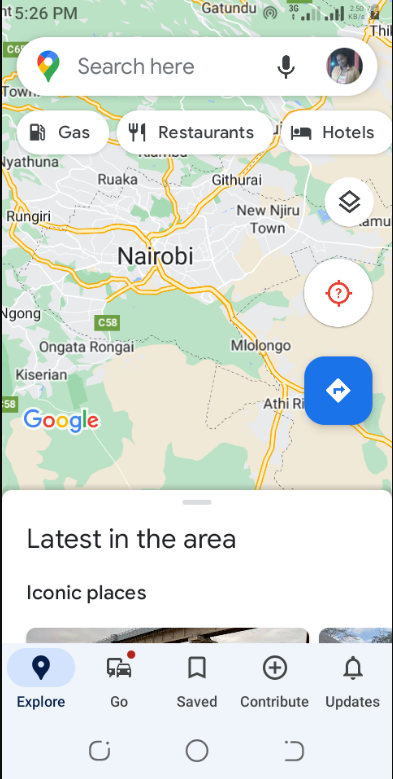The image is a screen capture from a mobile device displaying a map. The upper half of the screen is dominated by the map, which features various colors and patterns in green, cream, and light gray, representing different areas and landmarks. At the center of the map, the word "Nairobi" is prominently displayed in large black text, indicating the city's name. Surrounding Nairobi, there are additional locations also marked in black text, highlighting other key areas on the map.

At the top of the screen, there is a search bar with the Google Maps location icon on the left side, embedded in the white background of the search bar. On the right side of the search bar, there's a circular profile picture belonging to a user.

The bottom half of the image transitions into a white background, where text is displayed. The heading "Latest in the area" appears in black text, followed by another line of text underneath that reads "Iconic places," indicating categories or sections providing information about notable locations within the area.